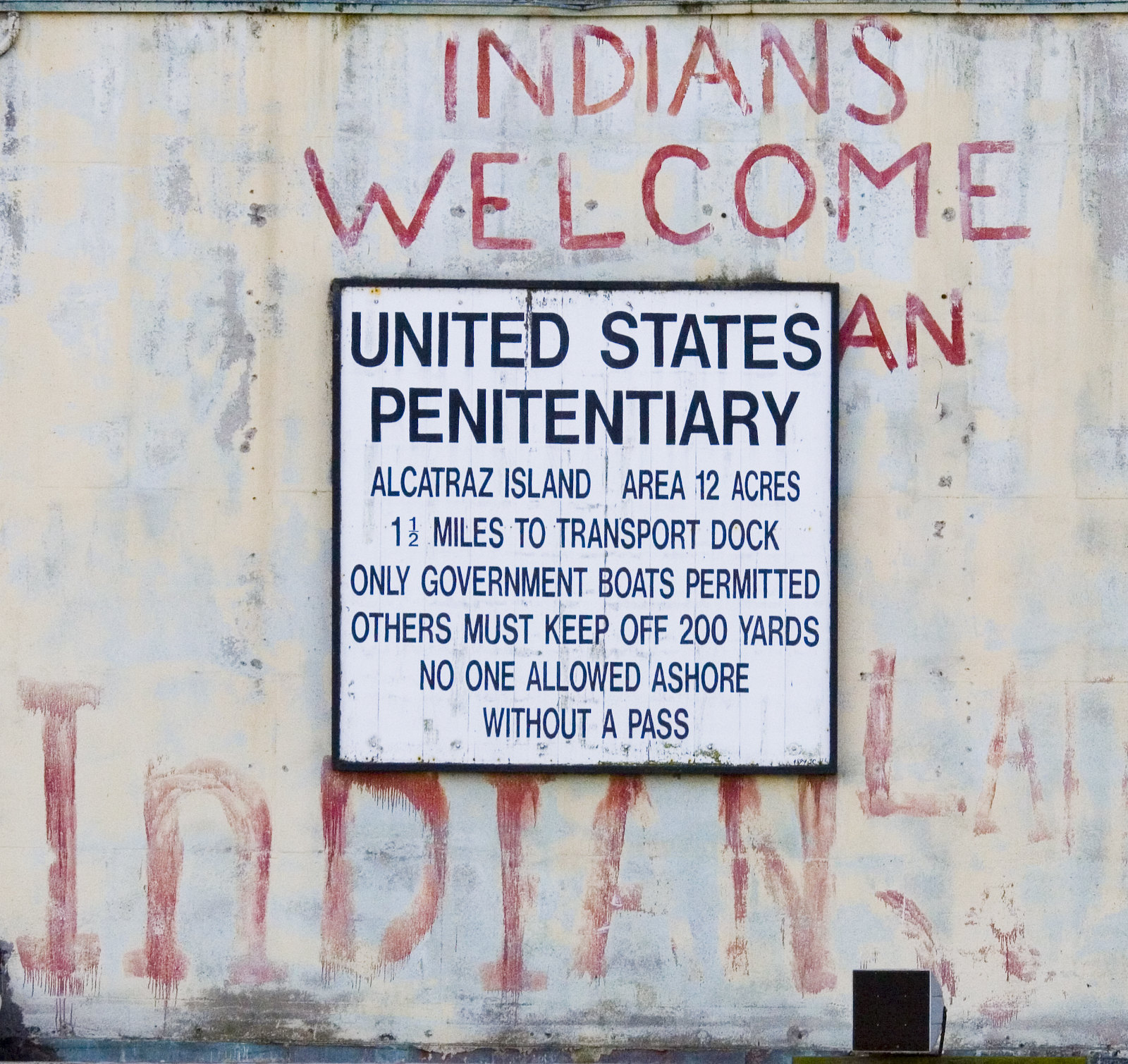The image depicts an aged, weather-beaten wall with a mixture of light yellow and gray colors, featuring extensive peeling paint and spots of rust towards the top. Prominently displayed in the center is a sign with a distressed white background outlined by a black border. The sign reads: "United States Penitentiary, Alcatraz Island, area 12 acres, one and a half miles to transport dock. Only government boats permitted. Others must keep off 200 yards. No one allowed ashore without a pass." Above this sign, in red ink, the wall is marked with the phrase "Indians Welcome," and below it, partially obscured by the sign, are the letters "A" and further down "Indian" followed by "LA" with additional letters that have been largely washed away. In the bottom right corner of the image, there is a small, gray-cased spotlight with a black center, angled slightly towards the left.